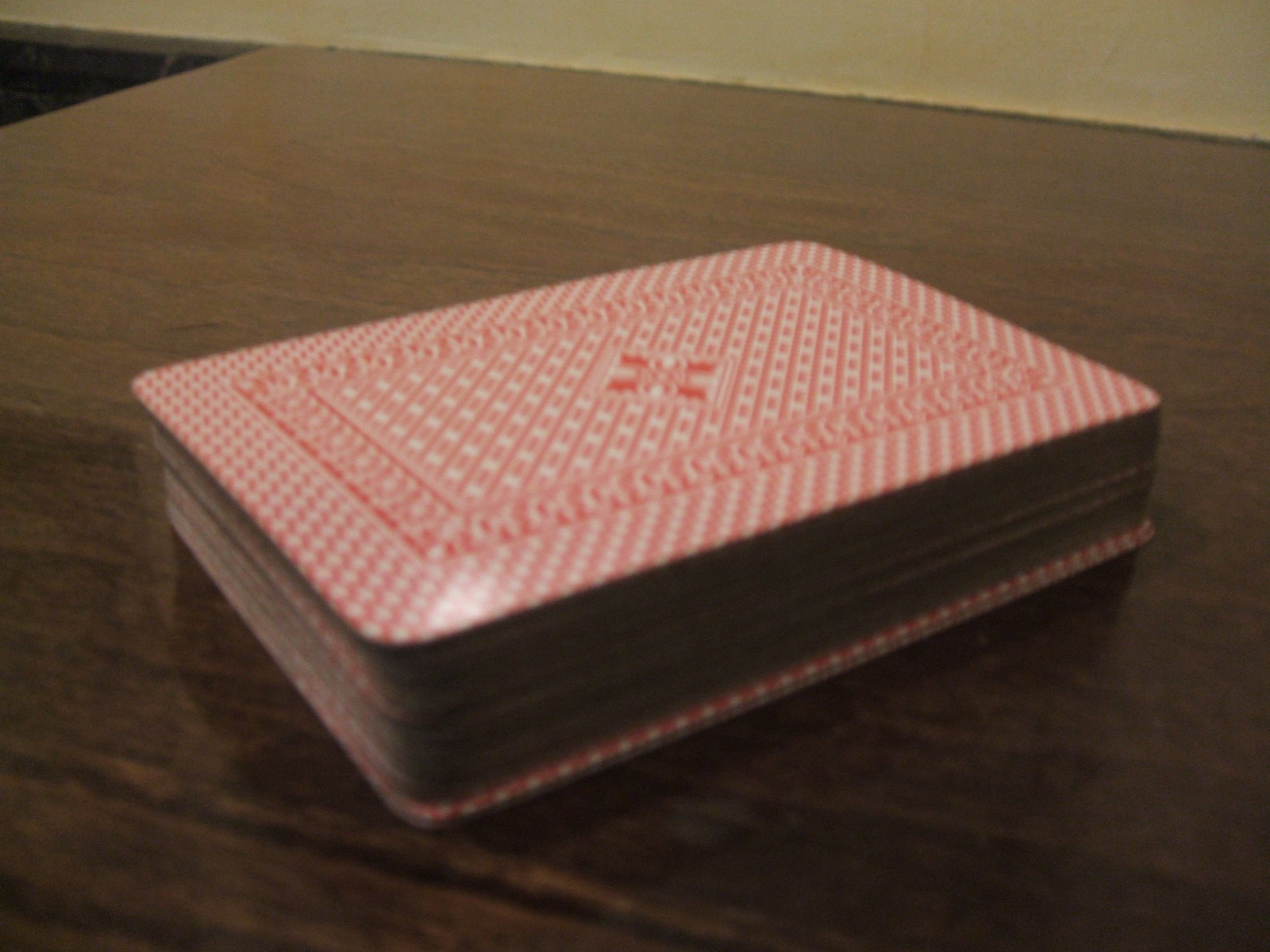This close-up photograph captures the detailed textures and colors of a deck of cards resting on a brown wooden tabletop. The shot is taken from a low angle, slightly above the deck, highlighting its orientation from the lower left to the upper right corner of the frame. The cards are neatly stacked, with gray edges visible and the long side of the deck more shaded, creating a sense of depth. The back of the cards features a striking red and white design with three or four repeating patterns. A subtle reflection of a bright light can be seen on the lower left corner of the deck, glinting off the glossy surface of the cards. In the background, a greenish wall suggests that the table is positioned either against or jutting out from it, adding to the cozy, indoor atmosphere. The photograph effectively contrasts the intricate details of the deck with the simplicity of its wooden and painted surroundings.